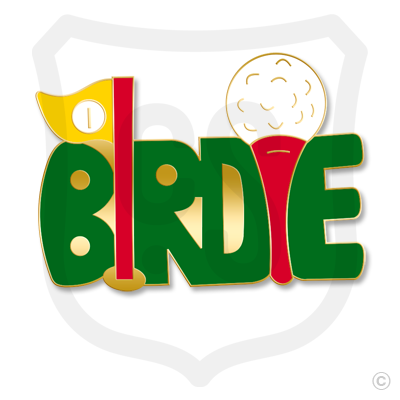The image features the word "BIRDIE" in a curved, bold font, with the letters B, R, D, and E presented in bright green, outlined in gold. The first 'I' is creatively replaced by a golf pin with a yellow flag that has a white circle and a yellow '1' on it; the pin is red with a gold base. The second 'I' is substituted by a white golf ball perched on top of a red tee, outlined in gold. The background showcases a very light gray shield resembling a highway sign, adding an interesting contrasting element. Additionally, there is a grayscale copyright symbol located in the bottom right corner, subtly blending into the white backdrop.